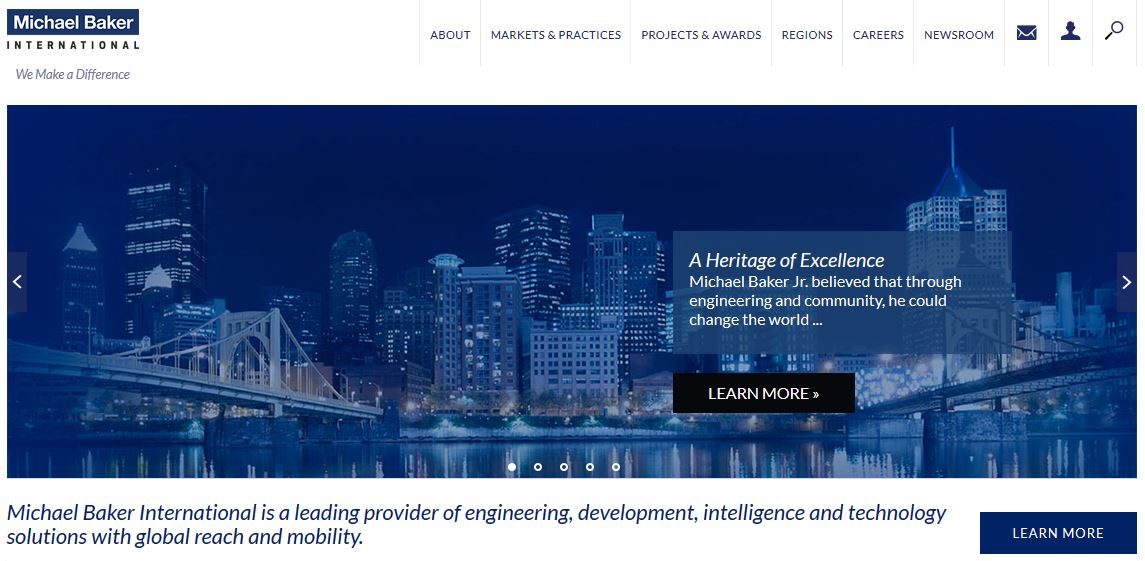The image features a blue-tinted photograph of a bustling cityscape dominated by a cluster of mid-sized buildings. A serene river cuts through the urban environment, flanked by two distinct bridges on the left and right. At the heart of the waterway lies a central dock, adding to the dynamic scene. 

At the top of the image, the text "Michael Baker International: We Make a Difference" is prominently displayed. Below this header, a navigation menu offers links to various sections including About, Markets & Practices, Projects & Awards, Regions, Careers, and Newsroom. Additional icons for email, search, and user profile are also visible. 

Further down, the image is overlaid with the slogan "Michael Baker International: The Leading Provider of Engineering, Development, Intelligence, and Technology Solutions with Global Reach and Mobility," accompanied by a blue "Learn More" button.

At the bottom, another statement appears, celebrating the organization's legacy: "The Heritage of Excellence: Michael Baker Jr. believed that through engineering a community, he could change the world," along with a black "Learn More" button.